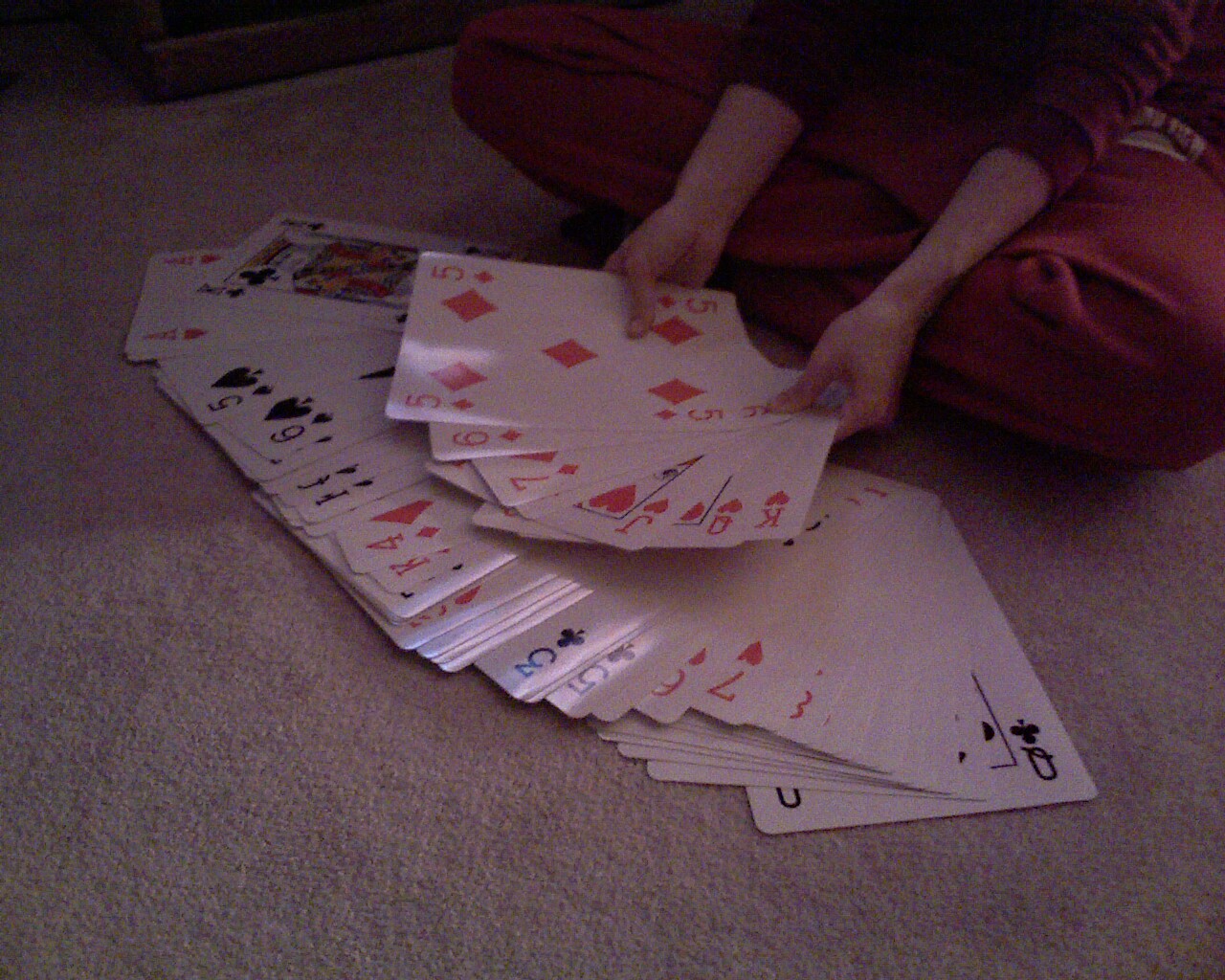In the photograph, a young girl is captured sitting cross-legged on a beige carpet, likely in a cozy lounge or sitting room. She wraps a red blanket snugly around her legs, juxtaposing her dark maroon sweater, which has its sleeves pushed up. Around her, a deck of unusually large cards is sprawled out on the carpet. Each card is almost the size of an A4 sheet of paper and appears to be laminated, giving them a glossy, durable finish. The oversized cards, perhaps made for a special project or as a unique gift, add a playful and intriguing element to the scene.